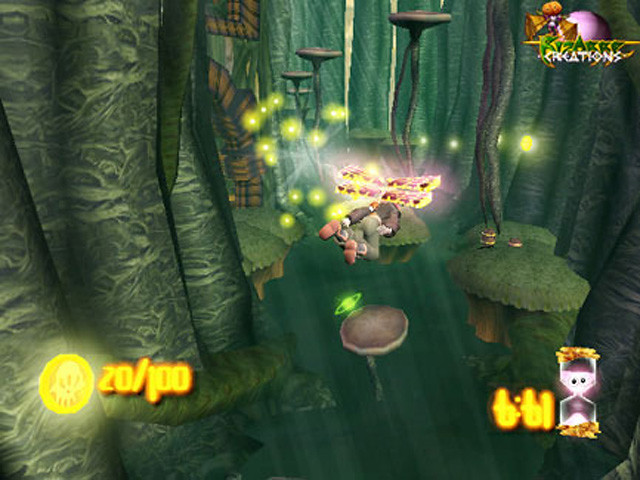This computer-generated image depicts an artfully designed scene from a retro-style video game. The background is enveloped in rich green hues, resembling a dense curtain of vines cascading down the screen, enhancing the game's nostalgic aesthetic. Scattered throughout the airspace are floating islands, some shaped like verdant patches of land and others resembling whimsical mushroom caps. Hovering amidst these suspended platforms is a humanoid character with delicate, transparent dragonfly wings, gracefully navigating the fantastical environment. Illuminating the scene are numerous glowing orbs in shades of green and yellow, adding a mystical quality to the ambiance. In the bottom-left corner, there's an overlay featuring a white skull emblazoned within a yellow circle, adjacent to a series of numerical indicators, indicative of typical in-game information displays or player stats.